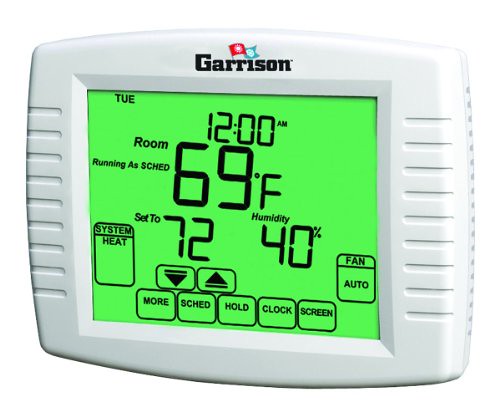In this image, there is a close-up of a digital thermostat. The thermostat is predominantly white with a green-lit screen displaying various details. The brand name "Garrison" is prominently printed in black ink at the top of the device. Notably, there are two small flags situated above the letters "R" and "I"; one flag is red, and the other is blue.

The screen is filled with information starting from the top, where the current day, Tuesday, is displayed alongside the current time, which is 12:00 AM. Below this, the thermostat shows the room temperature, which is 69°F. The system mode is indicated as 'Heat,' and the fan mode is set to 'Auto,' suggesting that it operates automatically. Additionally, the screen shows the indoor humidity level at 40%.

At the bottom of the thermostat, there are several buttons labeled "More," "Schedule," "Hold," "Clock," and "Screen," providing various control options for the user.